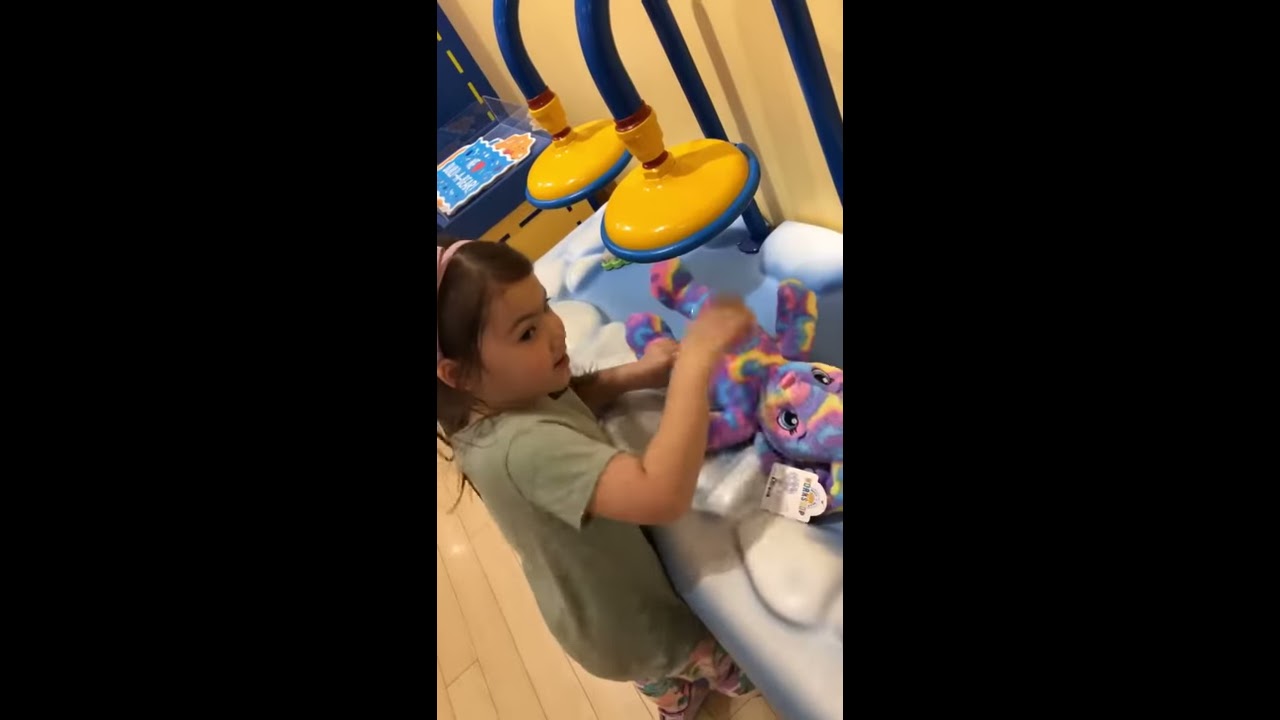A young girl, approximately 5 or 6 years old, is depicted joyfully playing with her toys in an indoor playground setting resembling a Build-A-Bear workshop. She has shoulder-length dark hair adorned with a pink headband and is dressed in an olive-grayish green shirt. The image is divided into three panels, with the central one showing her at an angle, requiring a slight tilt to the right to be upright. In the center panel, she stands in front of a yellow-walled toy counter with a hardwood floor reminiscent of a basketball court. Her arms are outstretched over a makeshift nurse's table, which features two descending lights and a multicolored, spring-themed stuffed bunny in shades of purple, blue, pink, and yellow. She smiles at the camera, holding her toy with evident delight, showcasing a playful and imaginative scene.